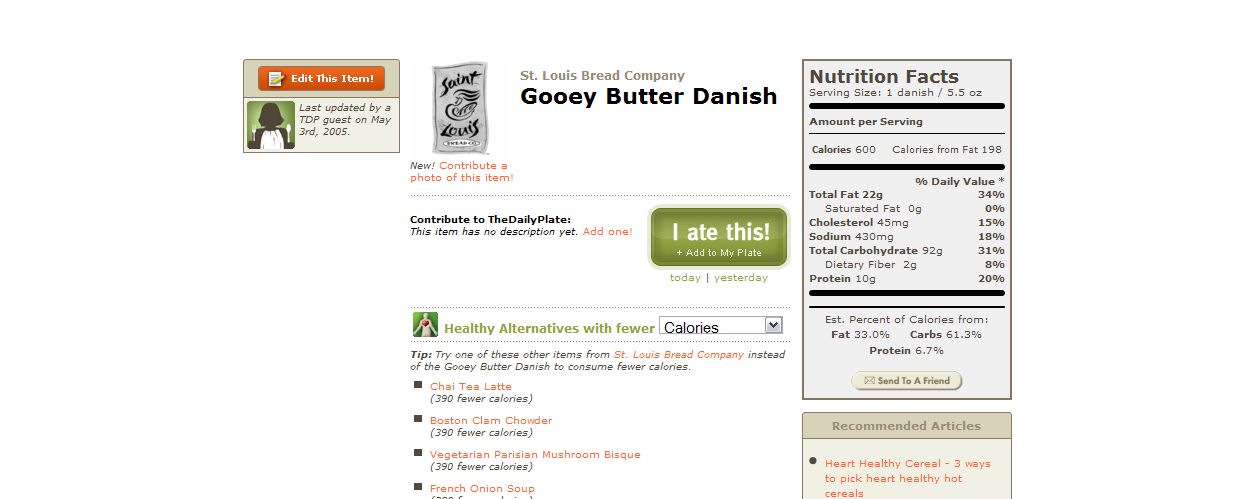The image is a screenshot of a food-related website or mobile application dedicated to tracking dietary intake. Prominently displayed in the middle upper section of the screen is the name of a food item, "Gwee Butter Danish." On the right side of the screen, there's a detailed nutrition facts panel providing specific health information about the Gwee Butter Danish. Further down on the right, there is an interactive button labeled "I Ate This," with an option underneath that says "Add to My Plate," suggesting a feature for users to log their food consumption and keep track of their dietary habits. At the bottom of the screenshot, a section titled "Healthy Alternatives with Fewer Calories" offers recommendations for lower-calorie options, helping users make healthier food choices. The overall layout and functionalities indicate that this is a comprehensive tool for those looking to manage their nutritional intake effectively.